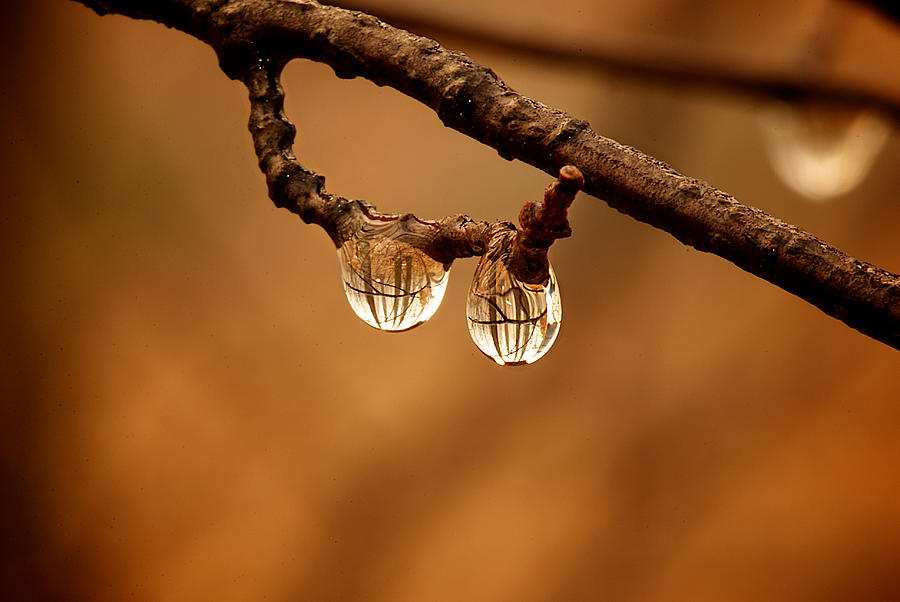This is a macro photograph featuring a dark brown, bumpy branch with two spherical water droplets hanging from a small section that loops backward. The water droplets, highly reflective and clear, capture intricate reflections of surrounding branches and some distinct orangish and white elements. The background, rendered in a beautiful, blurry brown and orangish-yellow gradient, adds depth to the composition. Another branch with a water droplet is partially visible in the blurred backdrop, enhancing the overall texture and warmth of the image. No text is present, focusing attention solely on the striking details of the bumpy branch and its shimmering water droplets.